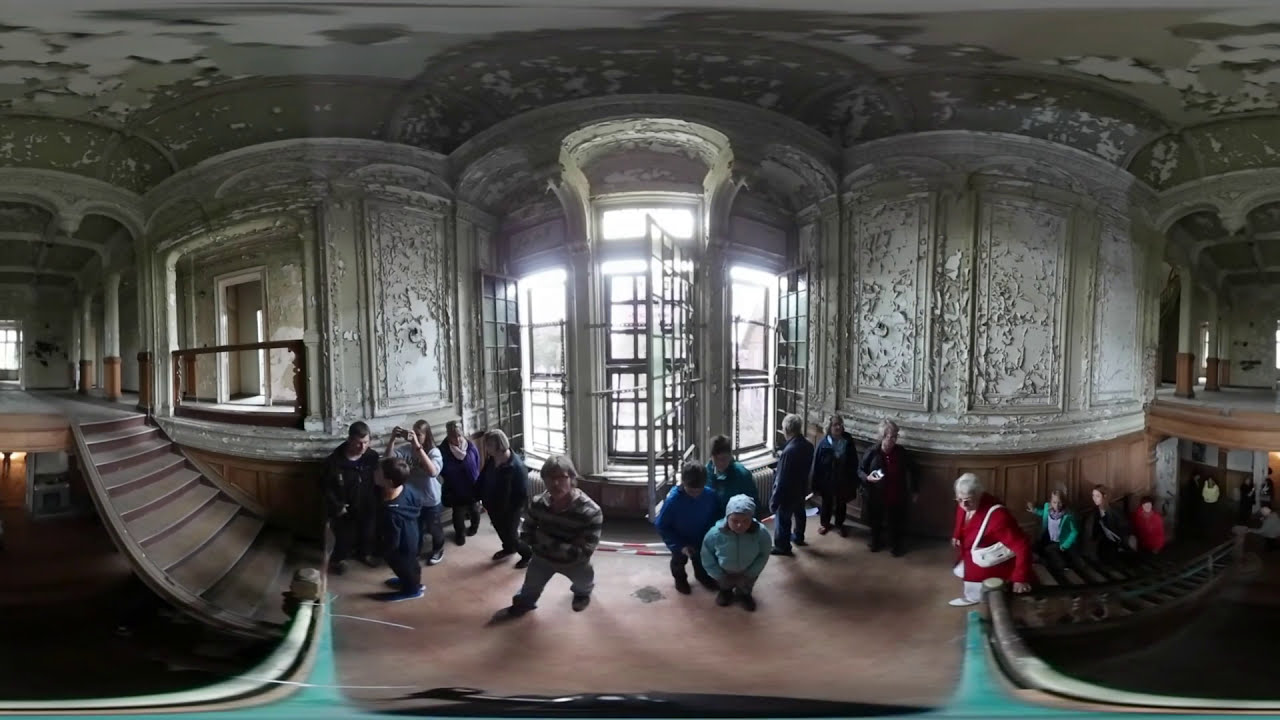This image captures the bustling interior of a grand, old museum or castle, where a crowd of visitors is taking a tour. The building has clearly stood the test of time, showcasing its dilapidated charm through cracked and deteriorating wallpaper, paint, and ceiling. The room is expansive, with ornate walls and impressive windows that extend nearly from floor to ceiling, featuring elegant rounded tops. 

In the center of the scene, a large window is under restoration, framed by wood paneling that is peeling away and crumbling, adding to the historical ambiance. People are gathered in front of the window, and many are ascending a curved wooden staircase, which leads to a landing and continues to the second story. These curved steps add a unique architectural element to the space.

Prominent among the visitors, some individuals stand out due to their colorful attire, including a woman in a striking red outfit and others dressed in green and black. The floor beneath them is a blend of tan and pinkish hues, possibly carpeted or hardwood. This picturesque setting, with its peeling walls and architectural elegance, draws numerous visitors who are keen to explore and experience the historical and cultural essence of this remarkable, aged building.